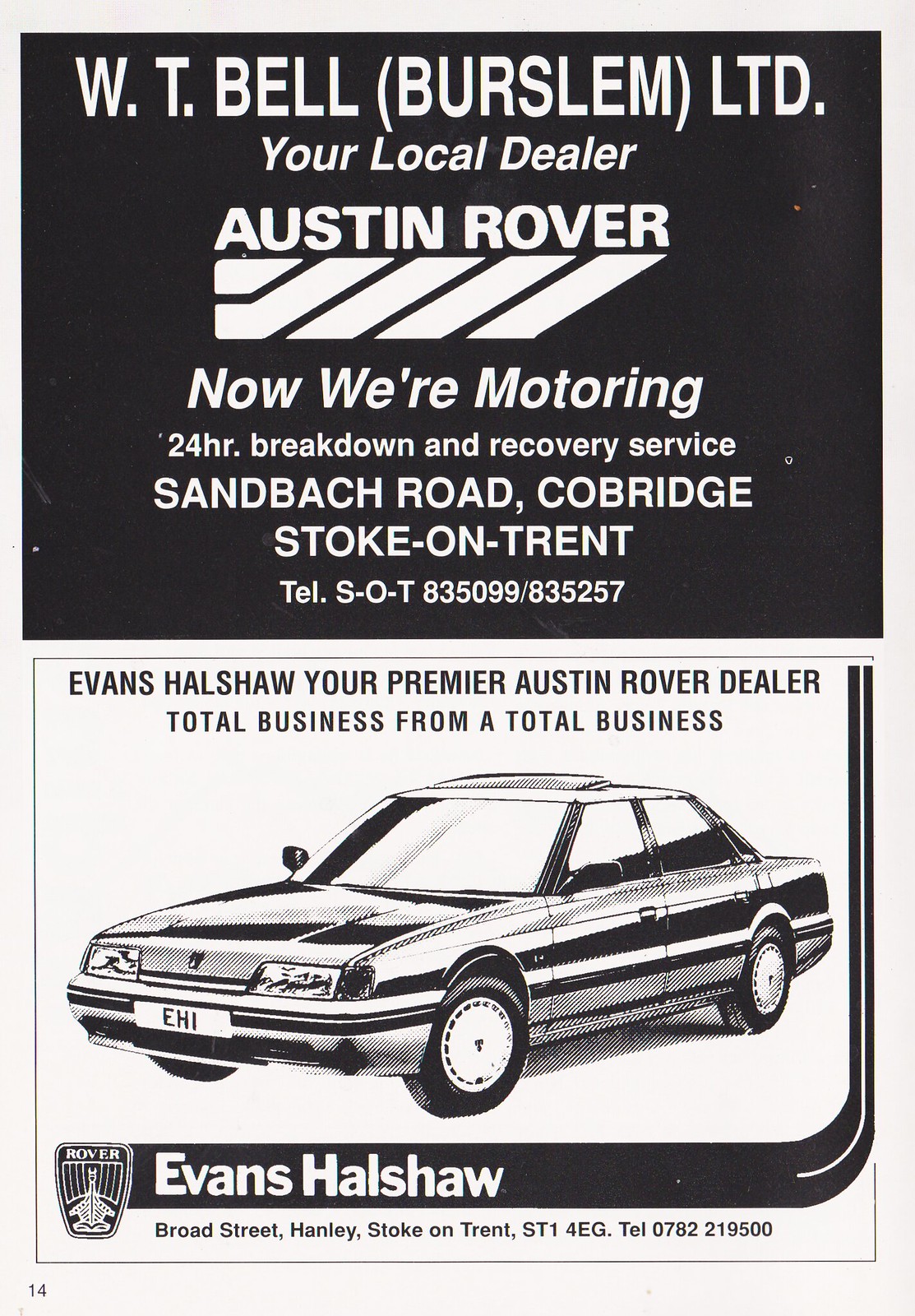This magazine advertisement for a car dealership is split into two distinct sections. The top section features a striking black background with white text that reads: "WT Bell, Burslem Limited, your local dealer. Austin Rover, now we're motoring. 24-hour breakdown recovery service. Sandbach Road, Cobridge, Stoke-on-Trent. Tel: SOT 835099/835257." Beneath this, the second section displays a white background with a thin black border, prominently featuring a black-and-white, hand-drawn image of a two-door car facing left. Above the car, in black text, it reads: "Evans Halshaw, your premier Austin Rover dealer. Total business from a total business." Additional text at the bottom right specifies Evans Halshaw's location as "Broad Street, Hainley, Stoke-on-Trent, ST1 4EG," with the contact number "Tel: 0782 219500." The bottom left corner of this section also showcases a small number "14", giving the ad a neat, organized appearance suitable for its magazine format.